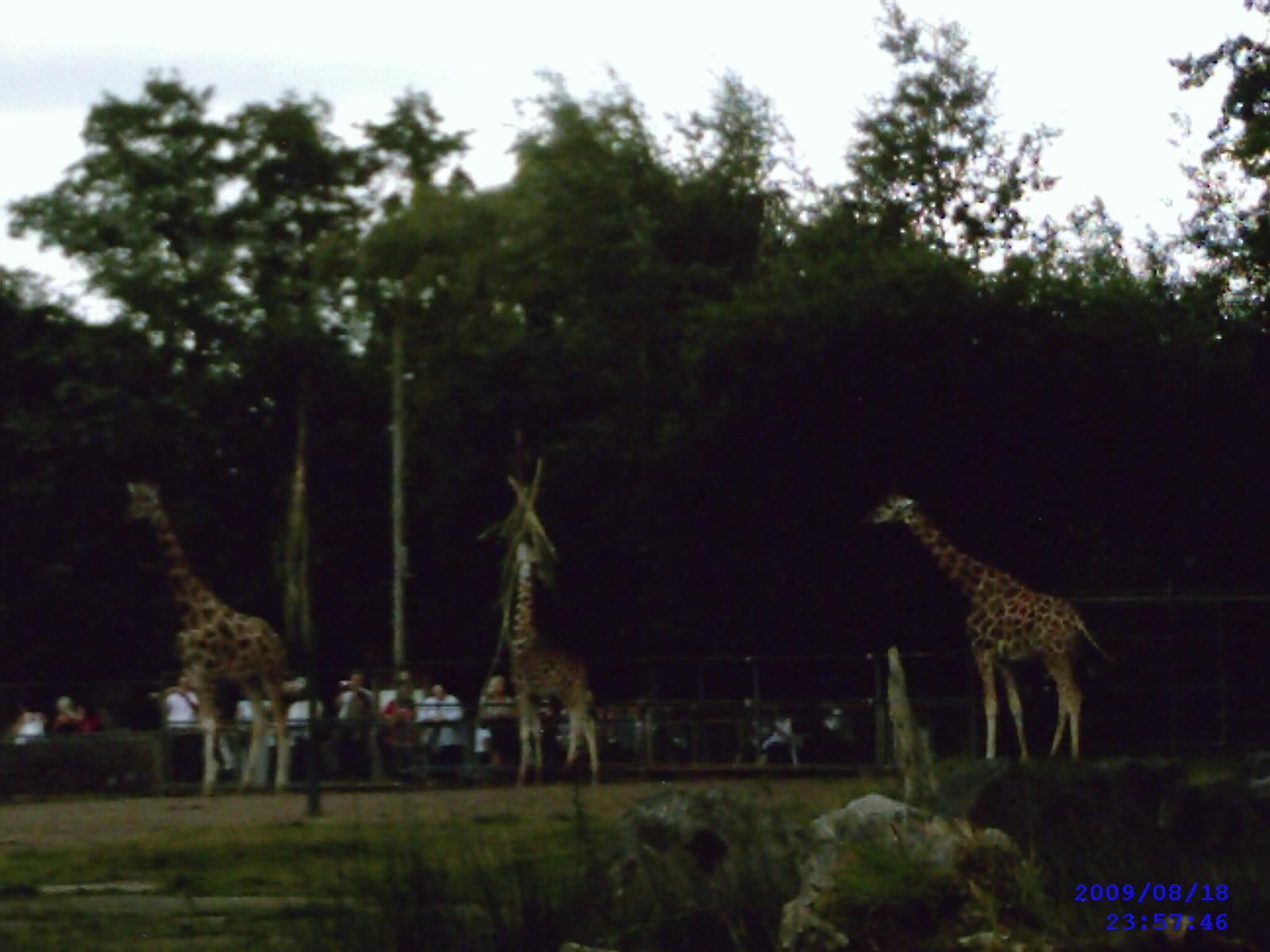In this poorly focused and underexposed photograph, three giraffes are captured in a dark, outdoor zoo enclosure. The giraffes, with their distinctive long necks, are somewhat hidden against a backdrop of dark trees. Above the trees, the sky appears bright white or very light blue, contrasting sharply with the overall darkness of the image. In the foreground, patches of grass and rocks can be seen, adding to the natural setting. Behind the giraffes stands a fence with people gathered on the other side, observing the animals. A light post is also visible near the fence. Notably, a date and time stamp in blue lettering is present at the bottom right corner, indicating the photograph was taken on August 18, 2009, at 23:57:46. The overall scene suggests the image could have been taken at dusk.